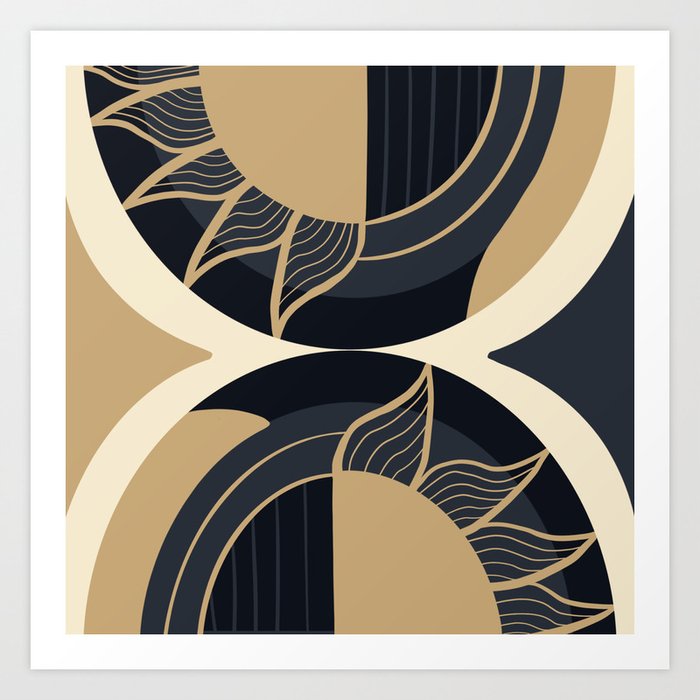The artwork is a computer-generated piece featuring two semicircles placed one above the other, almost mirrored but oriented in opposite directions. Each semicircle is divided into two distinct patterns: one half exhibits a dark blue lined pattern while the other half displays a beige or tan color. The beige side includes curvy, petal-like rays or leaf patterns, with detailed small tan lines running through them, whereas the dark blue side remains stark and linear. The top semicircle has four and a half petals or rays extending from the beige half, while the bottom semicircle showcases a similar design but in reverse orientation. The entire composition is set against a gradient background shifting from gray to black, surrounded by a white border, followed by a shadow and a light gray outer frame, giving the image a framed, layered appearance.